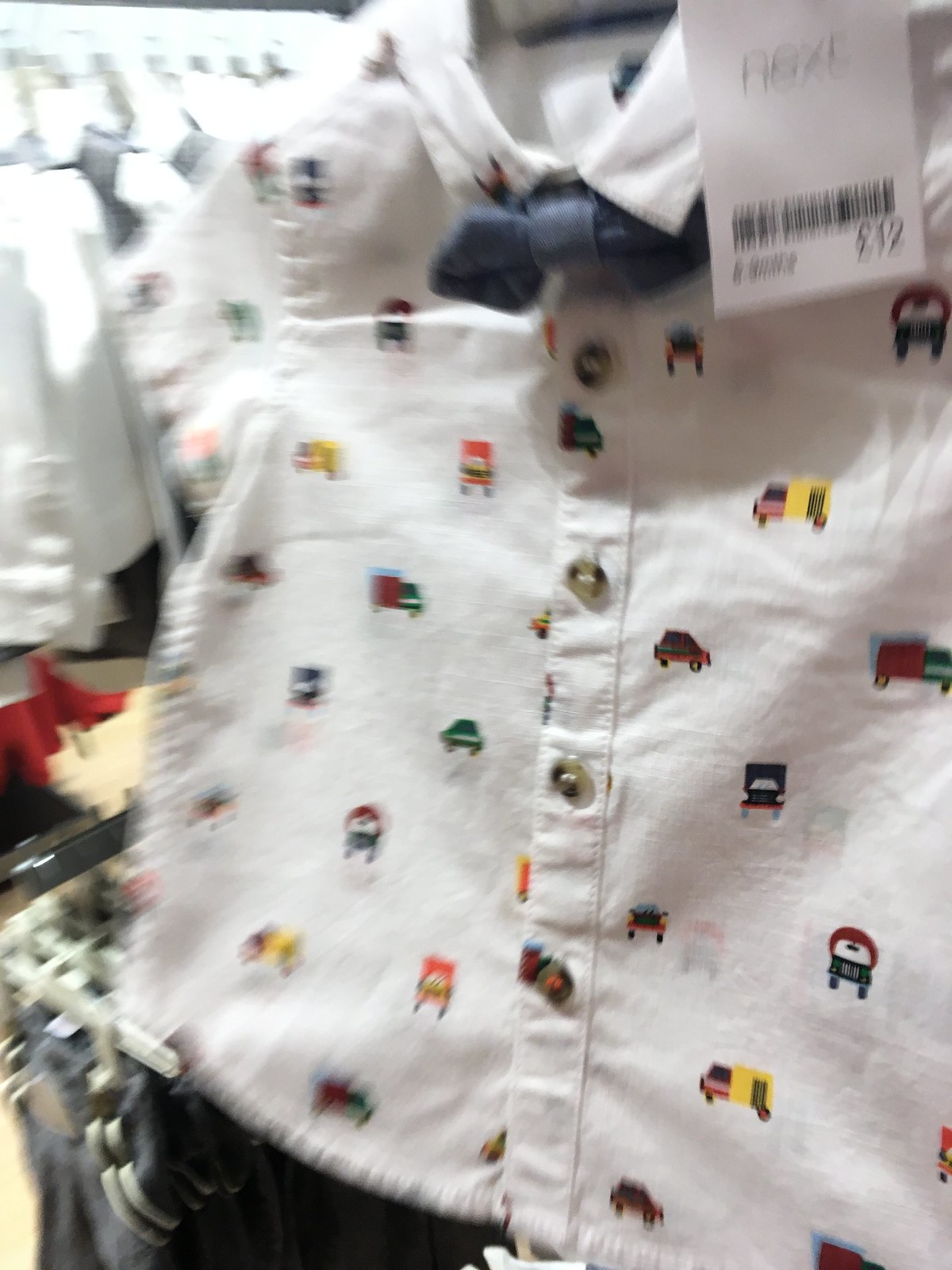This is a color photograph taken indoors, specifically inside a well-lit store, depicting a toddler boy's shirt prominently displayed. The shirt is white and adorned with small, multicolored images of various automobiles, such as cars, trucks, and buses, scattered across the fabric. Attached to the shirt is a blue bowtie situated just below the collar. There's a white paper tag attached near the collar, bearing a barcode, the brand name NEXT, and the price of $12 (or possibly 12 British pounds considering the blurred text). Despite the photo being somewhat blurry, the brand tag and automobile prints are discernible. In the background, there is a haphazard array of other toddler clothing, also hanging on racks. Notably, in the bottom left corner, jeans are displayed on plastic hangers affixed to a black metal rack.